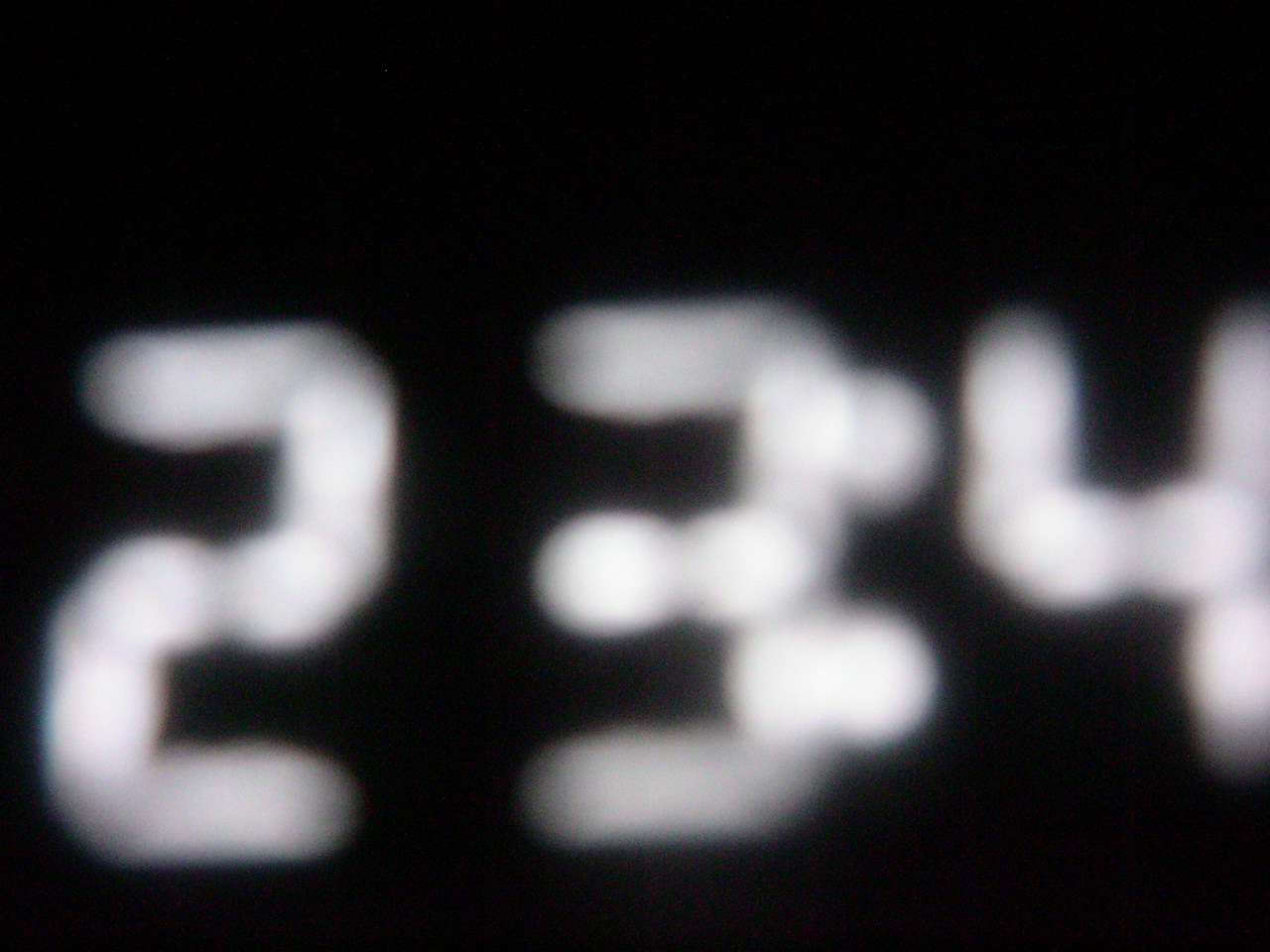Close-up, blurry image of an illuminated digital clock displaying the time. The background is completely black, accentuating the bright white digital numbers that dominate the frame. The visible digits are a "2," a "3," and a partially obscured colon, indicating the minutes are just out of view. The digit "3" and the colons appear slightly overlapped, possibly due to the angle of the photograph. The time displayed suggests it is 2300 hours and a few minutes past, though the exact minute is unclear.